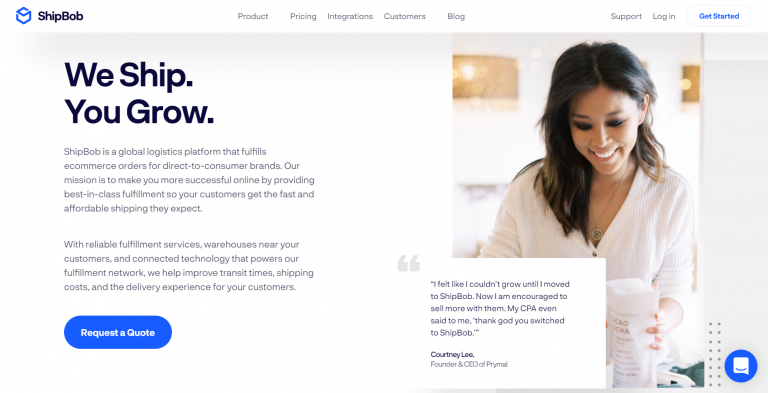This image is a detailed screenshot of a webpage from the website ShipBob. In the top left-hand corner, the company's logo, a blue outline of a three-dimensional box or cube, is prominently displayed. Adjacent to the logo, on the top right-hand side, are several navigation buttons: Support, Login, and Get Started.

Moving towards the center of the top section, there is a navigation bar featuring five clickable buttons labeled: Product, Pricing, Integrations, Customers, and Blog, arranged sequentially from left to right.

The main body of the page includes a bold, large title on the left that reads, "We Ship, You Grow." This is followed by a description detailing the website's shipping services. At the bottom left-hand corner of the page, there is a blue button with the text "Request a Quote," allowing users to easily request a quote for services.

On the right-hand side of the body, there is an image of a woman with dark hair and highlights, wearing a white top and looking downwards. The design and layout collectively emphasize the website's professional services and easy navigation.